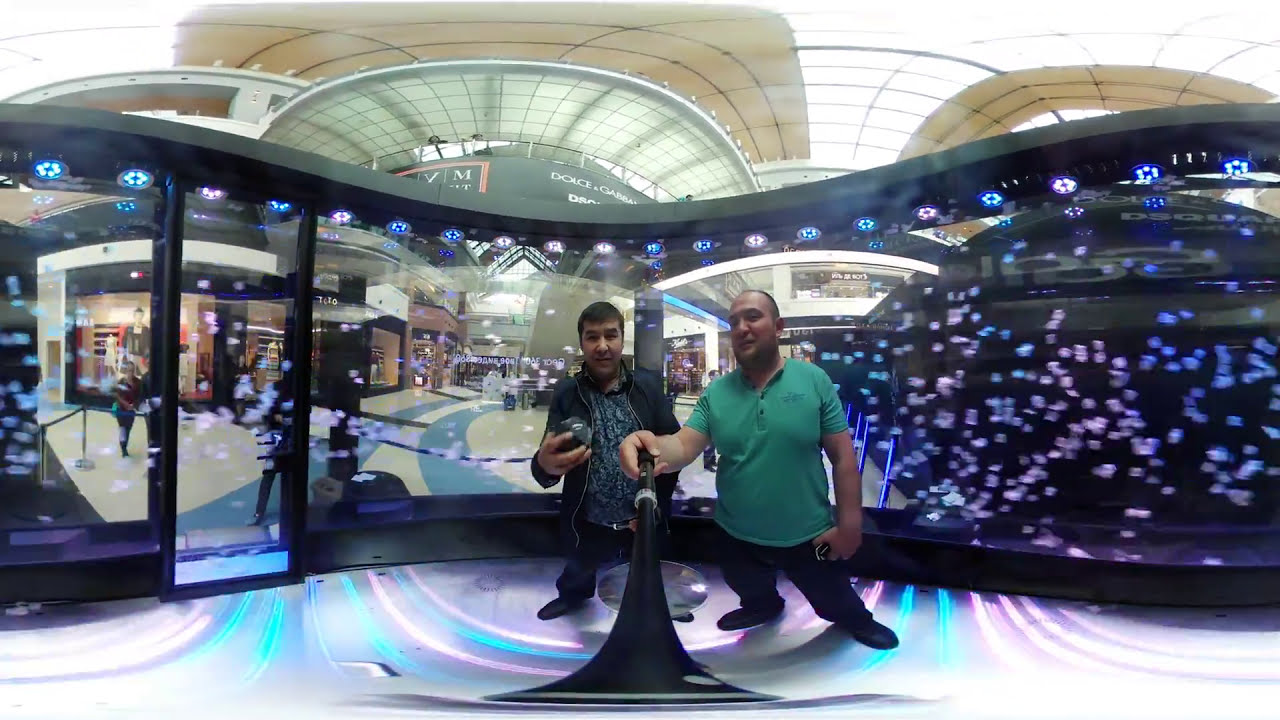This vibrant indoor image captures two men centered in a colorful room within a shopping mall. The man on the right, with short hair and wearing a green short-sleeve shirt paired with dark jeans, holds a long selfie stick with a phone mounted on its end, appearing to take a picture or video. The man on the left, slightly looking off-camera, has longer hair and is clad in a long-sleeve shirt with dark jeans, holding a ball-like object in his right hand. The room they stand in is lit with dynamic, color-shifting lights, primarily showcasing shades of pink, blue, and purple, with intricate lighting effects that seem to blend into the surroundings. This setting leads into an expansive mall area that features a variety of stores, including a prominent Dolce & Gabbana sign, and is bustling with people. The mall’s ceiling is notably tall with tan and transparent sections, allowing light to flood in, while the flooring presents a distinct blue and white curved pattern. The scene encapsulates the lively and colorful ambiance typical of a modern shopping mall during the day.